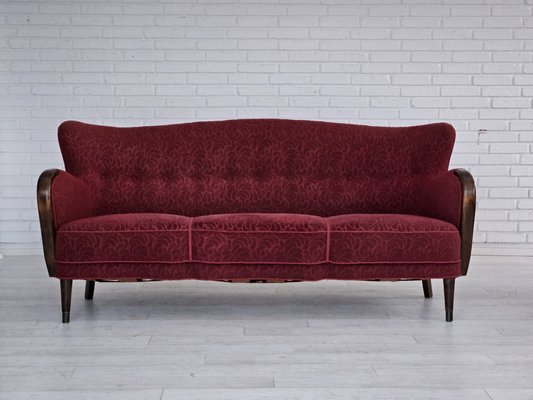This color photograph captures a luxurious antique-style burgundy sofa in the center of a minimalist white room. The sofa comfortably seats three people, featuring three distinct cushioned areas. It has a solid backrest, short wooden legs, and a dark wooden frame that includes wooden armrests. The burgundy upholstery is plush and has a subtle floral pattern formed by delicate curved lines. The sides of the sofa have a wingback design, adding to its gothic and vintage aesthetic.

The room's flooring appears to be white-painted wooden panels, aligned horizontally, creating an illusion of a wooden floor. The backdrop is a white brick wall, with the bricks running horizontally across. Shadows from the sofa fall subtly on the floor, giving the scene a touch of depth. Despite some uncertainty about its actual age, the sofa's intricate details and rich appearance suggest a piece that feels both classic and expensive.